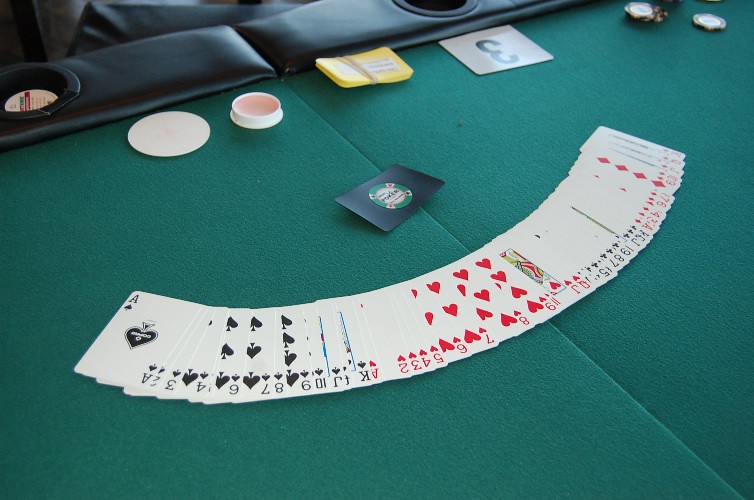In this detailed image, we can observe a blackjack dealer's table, characterized by its dark green velvety surface. A freshly opened deck of playing cards has been meticulously fanned out from left to right across the table. The cards are arranged in a perfect sequence, starting from the Ace in the center and proceeding outwards in descending order: 2 through 10, followed by Jack, Queen, and King. This flawless arrangement indicates a brand-new, unshuffled deck.

Below or above the deck of cards, there appears to be a business card, likely bearing the name of the establishment operating the blackjack table. Positioned slightly higher, there is a small plastic lip, which holds a tube of lip balm. To the right side of the table, a small stack of cards is secured together with a rubber band, and a placard displaying the number three is present in the top right corner. Nearby, some poker chips are also visible.

In the top left corner, we can see black, velvet armrest mitts, designed to provide comfort for the dealer as they manage and deal cards to the players, preventing fatigue. 

The image's primary focus is the honest display of the blackjack dealer’s table, with the perfectly fanned-out deck of cards, showcasing a trustworthy setup for the game.